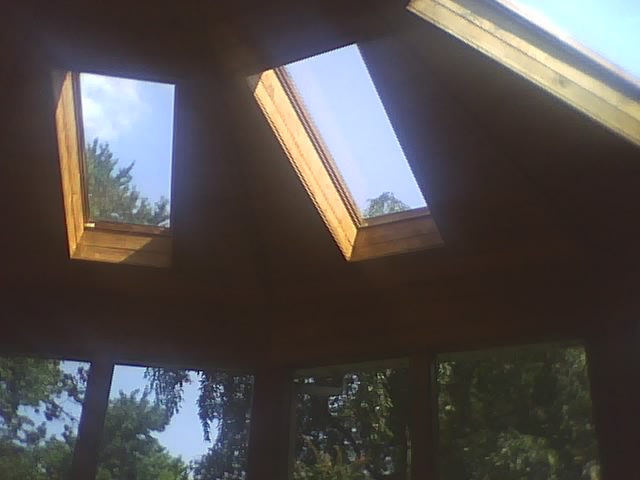The image captures an elegantly designed indoor room, completely adorned in beautiful wood, with a curved configuration. The ceiling, angled slightly upwards in the photo, features a series of deep, recessed rectangular skylights that follow the curve of the roof. These skylights provide glimpses of a bright blue sky dotted with white clouds and the lush greenery of trees and shrubs outside. The thick wooden sills around the skylights emphasize the robustness of the structure. Additionally, the room is surrounded by several windows that further frame the natural landscape outside, reinforcing the harmonious connection between the interior and the natural surroundings.